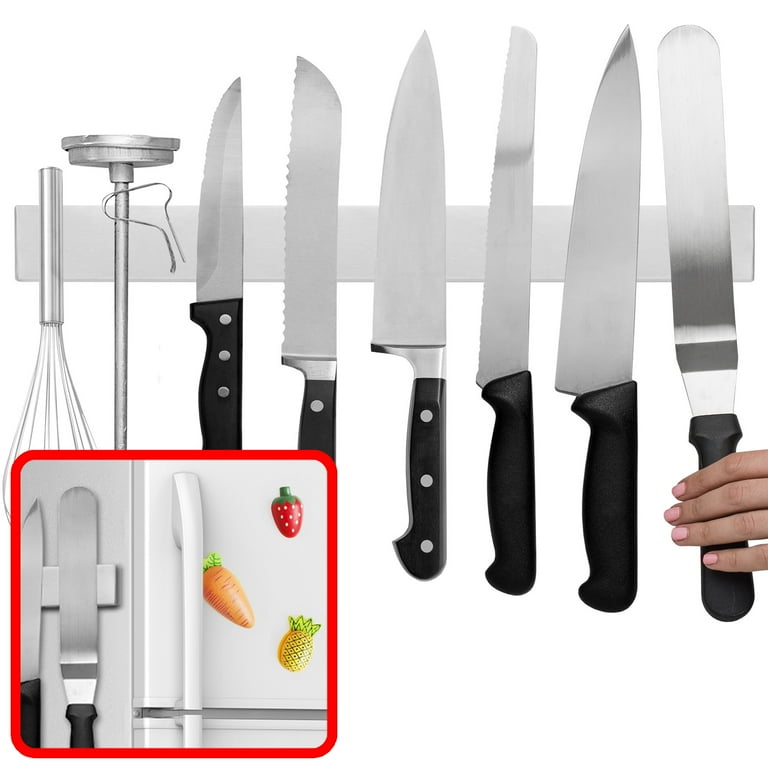In this detailed image, a set of kitchen tools is organized vertically on a stainless steel magnetic strip against a clean, white background. The collection includes a variety of knives with serrated and smooth edges, a thin and long spreader, a whisk, and a meat thermometer. Each tool has a black handle, and every blade and tool faces left. A person's hand grasps the handle of the spreader on the far right side of the picture. The main image is complemented by an inset photograph in the lower left corner, outlined in red, showing the magnetic strip attached to the side of a white refrigerator. This inset also displays colorful magnets shaped like a strawberry, carrot, and pineapple on the freezer door, further emphasizing the kitchen setting. The photograph appears edited, offering a clear and visually appealing presentation of the magnetic strip and its organization.